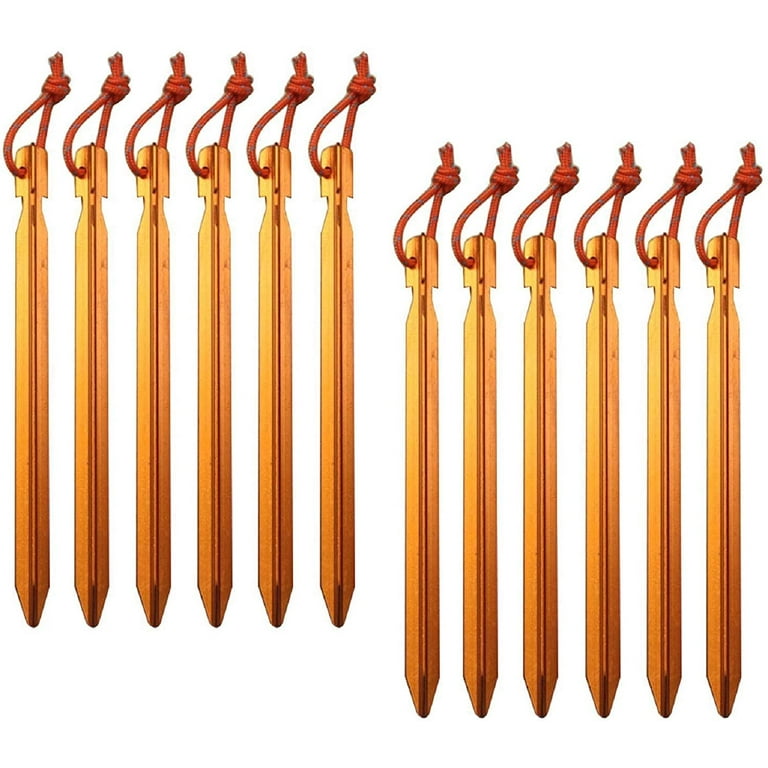The image depicts twelve pencil-shaped objects that appear to be wooden with a yellow exterior and a red line running vertically to the black pointed tip at the bottom, reminiscent of a pencil's graphite line. These objects are arranged in two neat vertical rows: the left row contains six items positioned slightly higher than the six in the right row, which hang slightly lower. Each object features a square-notch hole at the top through which a red thread is threaded and tied in a knot, resembling hanging pendants. Despite their pencil-like appearance, the metallic texture and the design details suggest they might serve a different purpose. The overall arrangement is precise, enhancing the visual impact of their aligned forms and consistent spacing, creating an impression of orderly and decorative display.